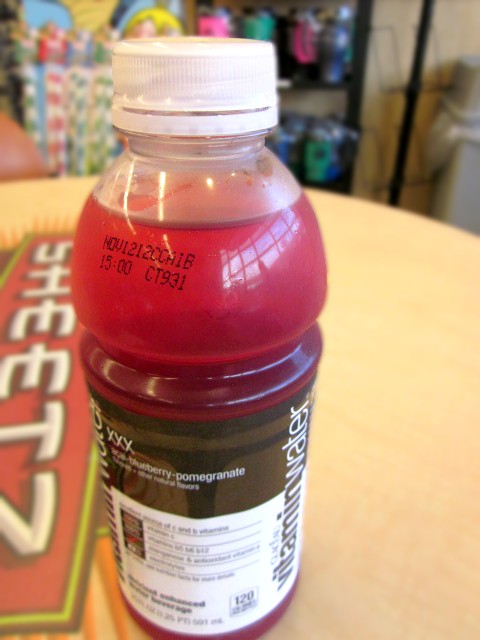This is a detailed image of a bottle of vitamin water, prominently positioned on a round, brown table. The bottle, filled with rich red liquid, sits front and center, slightly tilted to give a clear perspective of its contents. The vitamin water is of the strawberry pomegranate flavor. The top of the bottle features a white screw-off cap, beneath which is a transparent section of plastic showing the expiration date and batch information ("NOV 1212 CCA1B", "15-00", and "CT931") on the red liquid. The upper half of the bottle's label is green—displaying the brand name "vitamin water" in bold black and white letters along with three 'X' marks—while the lower half is white, containing nutritional facts in black lettering, although slightly blurry. Condensation on the bottle suggests it is cold and potentially opened, as it appears slightly less full. To the left of the bottle on the table is a red banner with white letters spelling "SHEETZ." In the background, on the left side above the table, are green and white striped belts, extending down to just behind the table, and higher up to the right is a brown ball with a black pole descending behind the table. The photograph, taken indoors, indicates it was snapped at a Sheetz restaurant.